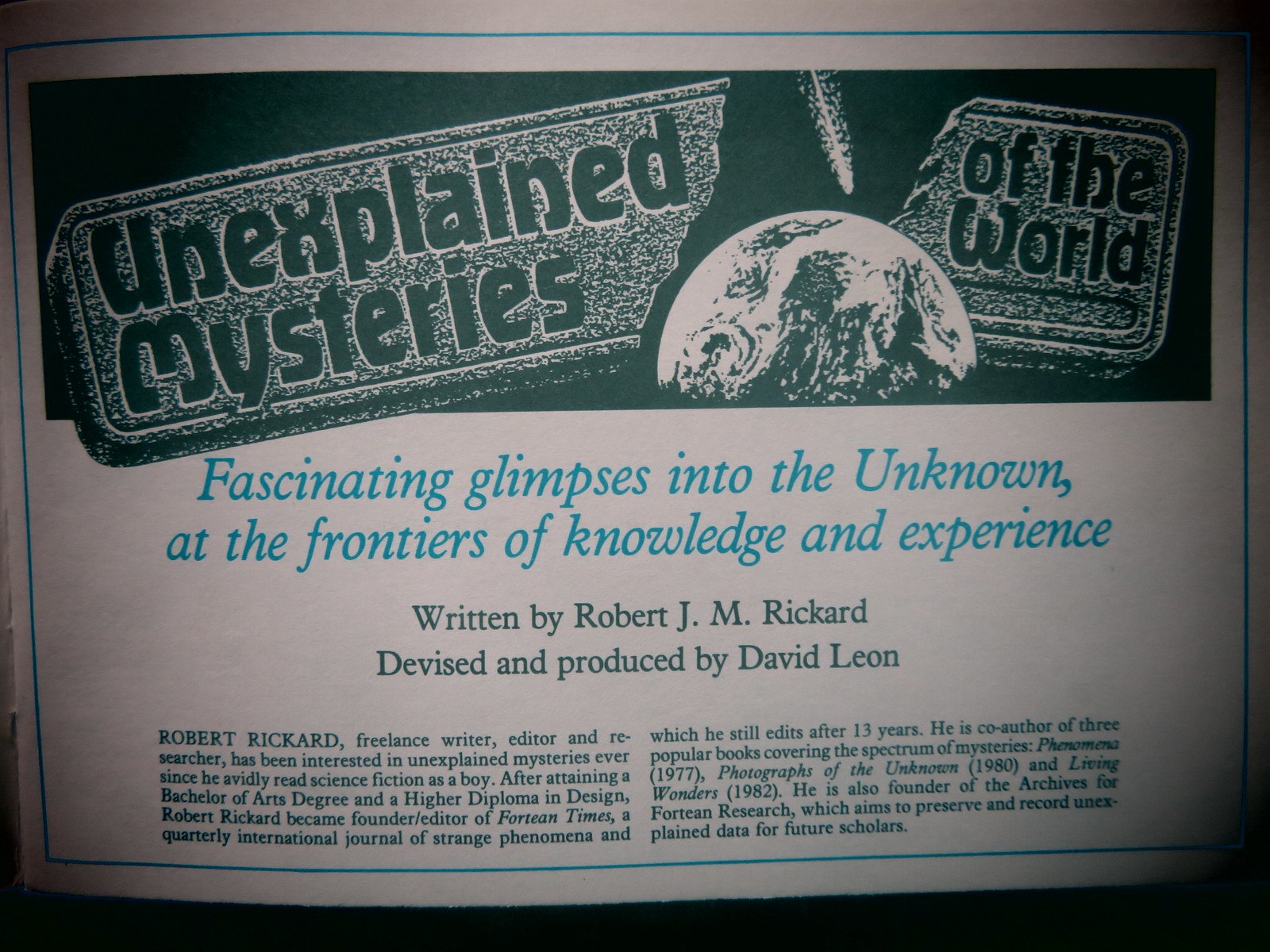The image appears to be a page from a book or a printed document, slightly bowed upwards as if the page is being turned. At the top of the page, there is a prominent black banner featuring an illustration of a cracked white stone overlaid on an image of the Earth, suggesting a comet heading towards the planet. This illustration is accompanied by large black text that reads "Unexplained Mysteries of the World." Beneath this banner, the title "Fascinating Glimpses into the Unknown at the Frontiers of Knowledge and Experience" is displayed in blue text against a white background. Further down, the text credits the work as written by Robert J. M. Ricard and devised and produced by David Leon, both in black font. The page is bordered by a thin blue line, adding a touch of detail to the layout. Below these credits, the text begins the article with an introduction to Robert J. M. Ricard: "Robert Ricard, freelance writer, editor, and researcher, has been interested in unexplained mysteries ever since he avidly read science fiction as a boy." The article then proceeds to provide more background information on Ricard.